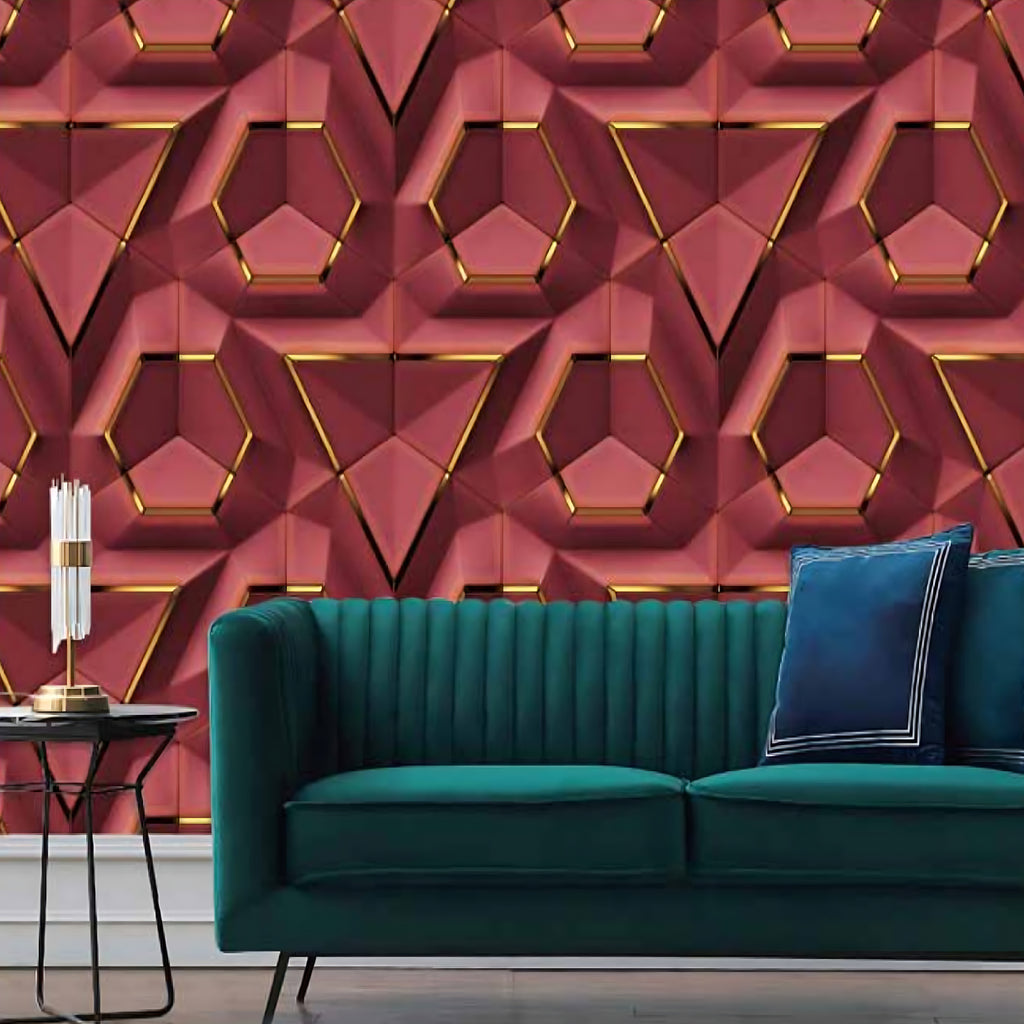This is a computer-generated mock-up of a living room interior. The room features a dark green mid-century modern sofa with clean lines, which is only partially visible on the right side of the image. On the sofa, there are blue decorative pillows. To the left of the sofa stands a round side table with a metallic lamp. The back wall of the room is predominantly red and decorated with golden geometric designs, including triangles and hexagonal patterns. The furniture, including the sofa and the table, has black legs, adding to the modern aesthetic of the space. Overall, the design is unique and visually striking.